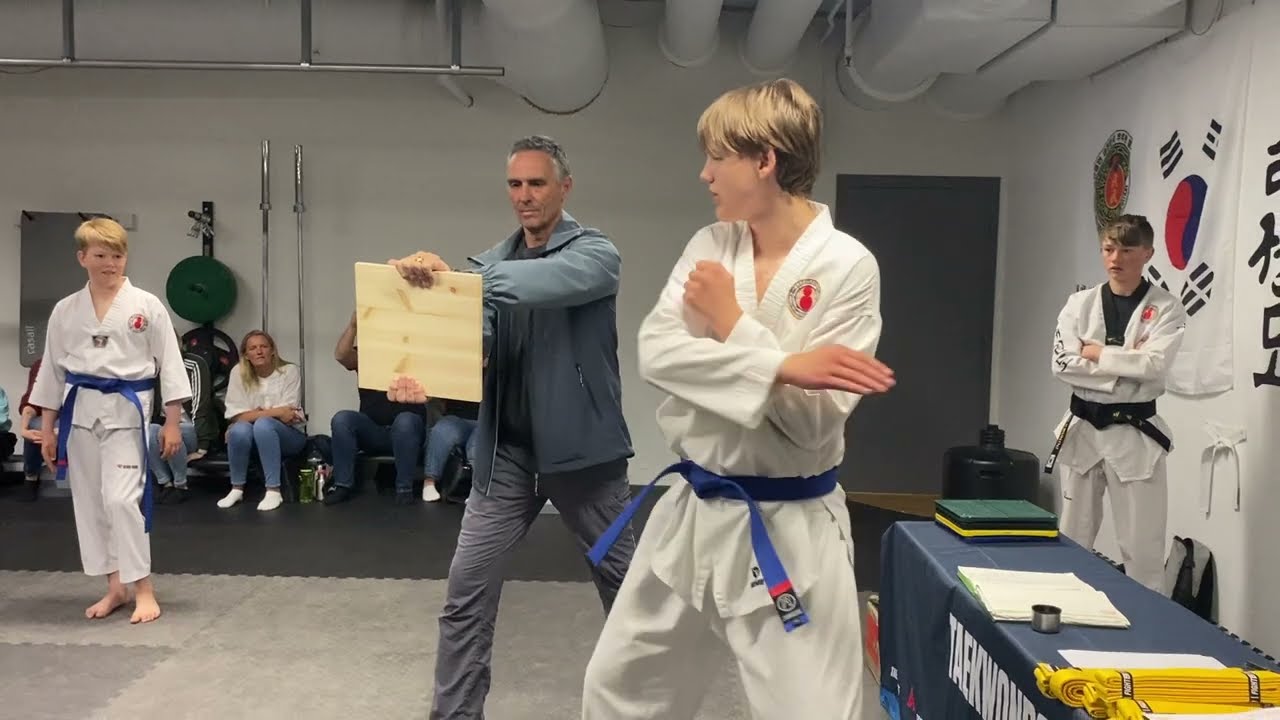The photograph captures an indoor scene at a martial arts dojo, likely a Taekwondo studio, evidenced by the Korean flag with a red and black yin-yang symbol hanging on a white wall to the right side of the image. The floor appears to be cement rather than padded. In the foreground stands a Caucasian teenage boy with blonde hair, dressed in a white gi and wearing a blue belt with a red stripe. He has his arms crossed in front of his chest and is intently focused on a wooden board held by an elderly man with gray hair, who is dressed in a blue jacket and gray pants. The boy appears to be preparing to break the board with a karate chop using his right hand. Behind him, two more boys in gis are observing; the one on the right has a black belt, and the one on the left has a blue belt. In the background, several adults, possibly parents, are seated and watching the demonstration. A table covered with a dark blue cloth that reads "Taekwondo" and holds some yellow belts and papers is positioned on the right side of the photo. Large pipes are visible at the top of the image, adding to the industrial feel of the dojo.